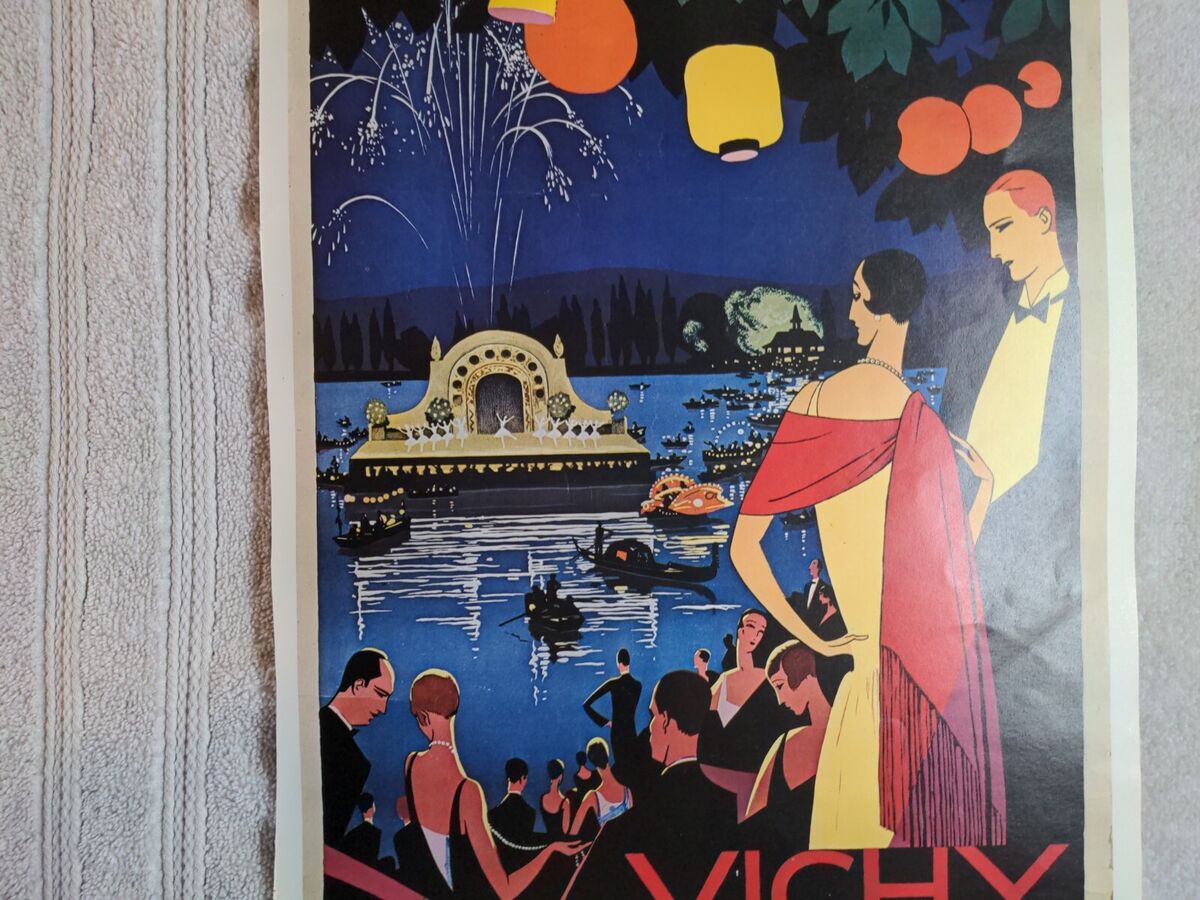This is an elegant and vibrant illustration, likely from a vintage travel poster or print from the early 20th century. The scene depicts a lively night by a lake, adorned with orange-yellow and red spherical Japanese lanterns hanging from trees and illuminating the festive ambiance. At the bottom, the word “Vichy” is prominently displayed, indicating the French town famous for its historical events and attractions.

In the foreground, a well-dressed crowd, reminiscent of the 1920s, is gathered. The women sport short, curled hairstyles with long scarves and elegant dresses, while the men are clad in tuxedos. They stand on the left side, observing the grand spectacle unfolding on the lake.

The centerpiece of the image is a floating stage on the water, surrounded by ornate boats, canoes, and gondolas operated by gondoliers. On this stage, approximately eleven women perform a graceful ballet under the illuminated sky filled with sparkling fireworks. Behind the stage, a large walled backdrop features a strikingly tall, arched opening.

In the background, gentle hills and a tree-lined shore frame this captivating scene, with the faint silhouette of a house visible on the distant bank. The harmonious blend of natural and human elements, tradition, and celebration makes this illustration a breathtaking representation of a festive night in Vichy.